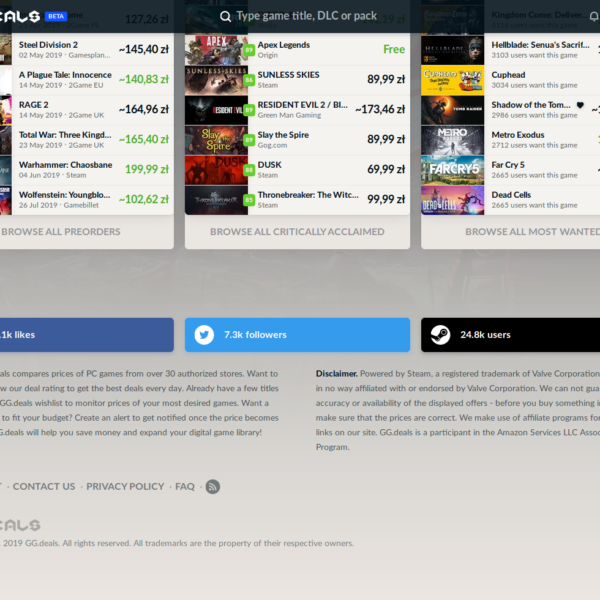The image depicts a partially visible website interface. At the top left corner, there is a partially cut-off logo displayed within a black banner. The logo is entirely white, with a small blue rectangle adjacent to it containing the word "Beta" in white text. Centrally located within this black banner is a search bar prompting users to type in a game title, DLC, or pack. 

To the right side of the banner, part of the content is cut off, but a bell notification icon is visible. Below the banner, the main content area shows various rectangular sections, each featuring images of games, their titles, release dates, and pricing information. The first row lists "Steel Division 2," released on May 2, 2019, with a game plan price marked as "14540ZT" in black text. Below it is "A Plague Tale: Innocence," released on May 14, 2019, priced at "140E3ZT" in green text. This pattern continues for three game listings in total.

Further down, there are large icon buttons for social media platforms, starting with Facebook and Twitter, followed by an unidentified black icon representing another social media site. The footer at the bottom of the page contains essential information such as disclaimers, contact details, address, and trademarks.